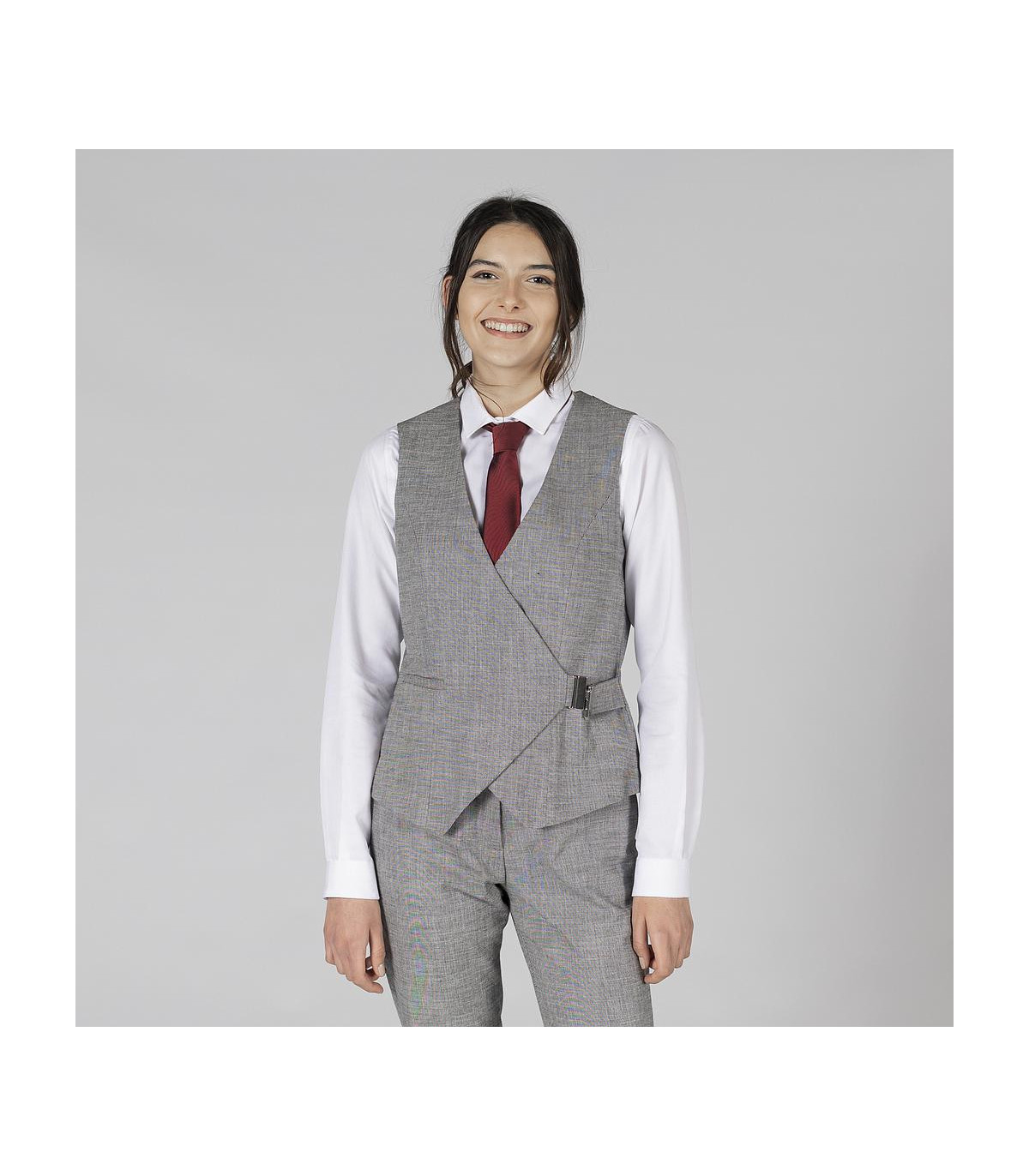In the image, a woman exudes elegance and sophistication, dressed in a meticulously tailored gray suit featuring a subtle pinstripe pattern that forms a slight checkered design. Her ensemble includes a sharply pressed, white or off-white shirt that contrasts beautifully with a striking red tie, adding a vibrant pop of color to her attire. The gray suit, which appears to be a slate gray, includes a distinguished vest that is fastened with a black clip and a belt that wraps around the back, reminiscent of classic formal wear detailing.

Her long, dark hair cascades gracefully, framing her face which is lit by a warm, genuine smile. She has light skin, dark expressive eyes, and well-defined dark eyebrows, enhancing her poised and polished appearance. The background is a light gray, subtly shaded by the ambient lighting, contributing to an overall soft and sophisticated atmosphere. Her attire and demeanor suggest that she is dressed for a formal event, radiating confidence and elegance.